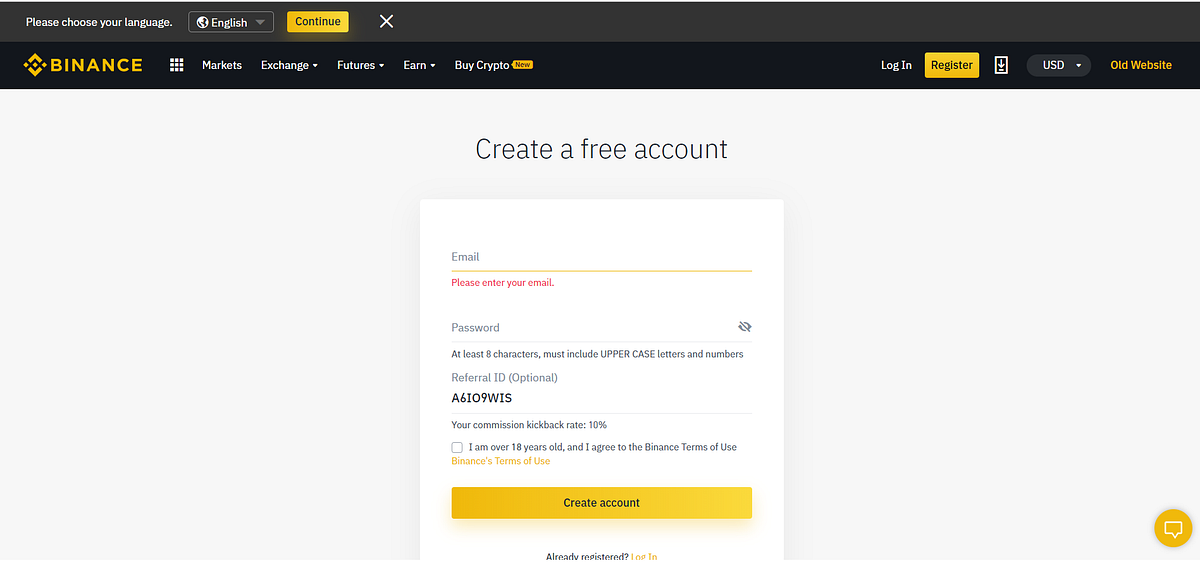A portion of our web page dedicated to account creation on Binance is depicted here. The top section features two black banners. The uppermost black banner prompts users to select their language, with "English" being the selected option, followed by a yellow "Continue" button and a "Close" button to the right. The second black banner displays the Binance logo and the word "Binance" in yellow. Adjacent to it are various navigation icons and tabs, including:

- A nine-box grid icon
- Tabs for "Markets," "Exchange" (with a down arrow for a dropdown menu), "Features" (with a dropdown arrow), "Earn" (with a dropdown arrow), and "Buy Crypto" highlighted with a yellow button
- Options for "Login" and "Register" (the latter being a yellow button)
- A download icon, a USD currency selector (with a dropdown arrow), and a link to the "Old Website" in yellow.

In the center of the page is a white form box titled "Create a Free Account." Within this form, the following details are required:

- An input field labeled "Please enter your email" for the user's email address
- A password field with a visibility toggle icon accompanied by a note that passwords must be at least eight characters long and include uppercase letters and numbers

Additionally, there's an optional section for entering a referral ID, with an example code "A6109WIS." Below that, the communication kickback rate is indicated as 10%. 

Users must check a box confirming they are over 18 years old and agree to the Binance Terms of Use, which include a link to the terms. At the bottom of the form, a yellow "Create Account" button is prominently displayed, alongside a link that reads "Already registered? Login" for returning users. Finally, a bot icon for asking questions is positioned at the bottom right of the page.